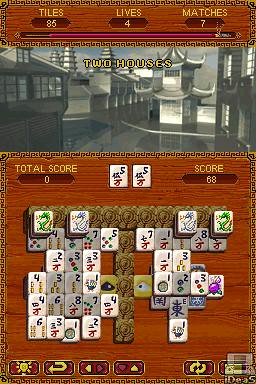This image is a screenshot from a Chinese-themed video game, likely designed for mobile devices given its shape and layout. The background features a reddish-brown, maroon hue, with traditional Chinese-style high-rise buildings depicted in grayscale, or a sepia-toned black and white, labeled "Two Houses" in yellow text. At the top of the screen, game statistics are displayed in yellow text: "Tiles: 85," "Lives: 4," and "Matches: 7." Below the top section, there's a purple bar crossing the width of the screen.

Central to the image are two white cards, each bearing the text "Total Score: 0." The area surrounding the cards is filled with rows of additional cards stacked vertically and horizontally. At the very bottom of the screen are control icons, likely including back and refresh buttons, along with various symbols displayed in purplish-red and yellow square boxes. The overall design indicates this image is from a Chinese-style card or tile-based game, with detailed, ornamental backgrounds complementing its traditional theme.